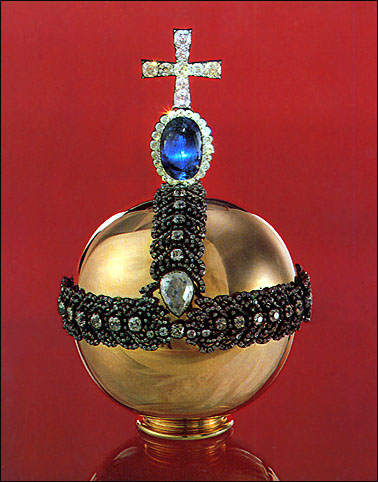The image features a regal, spherical gold object set against a red background, possibly a museum artifact or a piece of royal jewelry. The centerpiece of the object is a large, shiny blue stone, likely a sapphire, encircled by a ring of sparkling diamonds. Atop this sapphire sits a diamond-studded cross. Two straps, one horizontal and one vertical, adorned with metal stilettos, intersect around the circumference of the golden sphere. The intricate detailing and lavish use of precious stones suggest the piece's association with royalty or ceremonial significance, and it is displayed on a red table that complements the vibrant background.